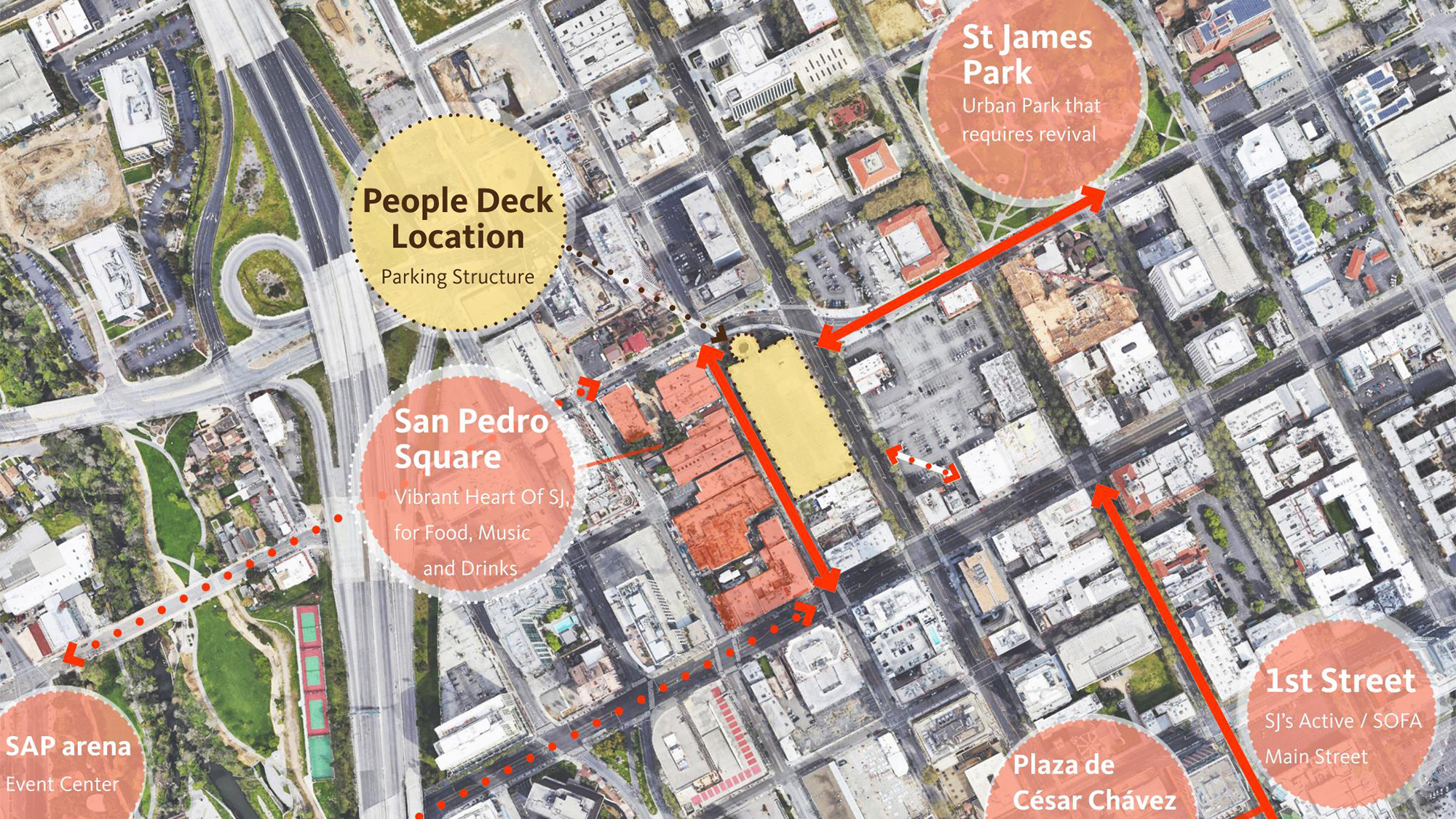The image is an overhead, almost Google Maps-like, aerial view of a city grid system highlighting key locations and routes. Central to the image is a large rectangular building shaded in yellow with a dotted arrow pointing to it, labeled as "People Deck location, parking structure." Surrounding this, multiple buildings are shaded in coral or salmon colors, identified as "San Pedro Square, vibrant heart of SJ for food, music, and drinks." The map also marks other important locations with red circles, including St. James Park, First Street, Plaza de Cesar Chavez, and SAP Arena. The roads are colored black with varying shades of gray for the buildings, and there are double-ended red arrows indicating movement up and down streets. The image aims to guide viewers through different routes and venues, likely for a specific event, by providing a detailed city planning layout.